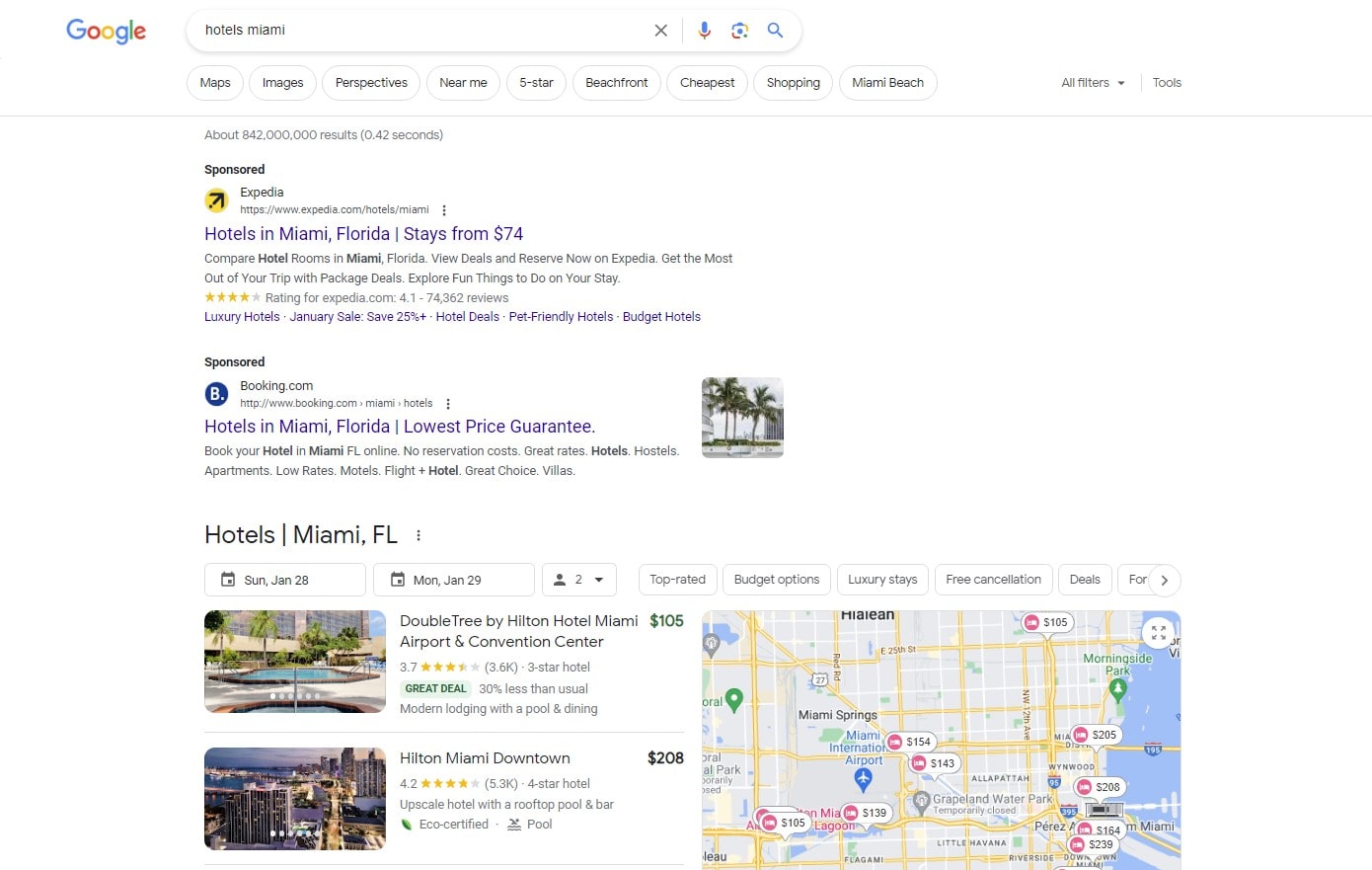A detailed image caption could be:

"In this Google search result for 'Hotels Miami,' the first two links are prominently marked as sponsored ads. The first link from Expedia offers stays in Miami, Florida starting from $74, while the second link from Booking.com promises the lowest price guarantee for hotels in Miami, complete with an inviting picture of palm trees. Beneath these links, there's an embedded section from Google allowing users to input their arrival and departure dates, specify the number of adults, and apply various filters such as 'Top Rated' and 'Budget Options.' Two hotel listings are visible: Doubletree by Hilton Hotel Miami at $105 per night, rated 3.7 stars out of 5 from 3,600 reviews and labeled as a 'great deal,' and Hilton Miami Downtown at $208 per night, sporting a superior 4.2-star rating and eco-certification. A small embedded map to the right shows that both hotels are close to each other near Miami Springs, with the nearby waterfront visible on the right side of the map."